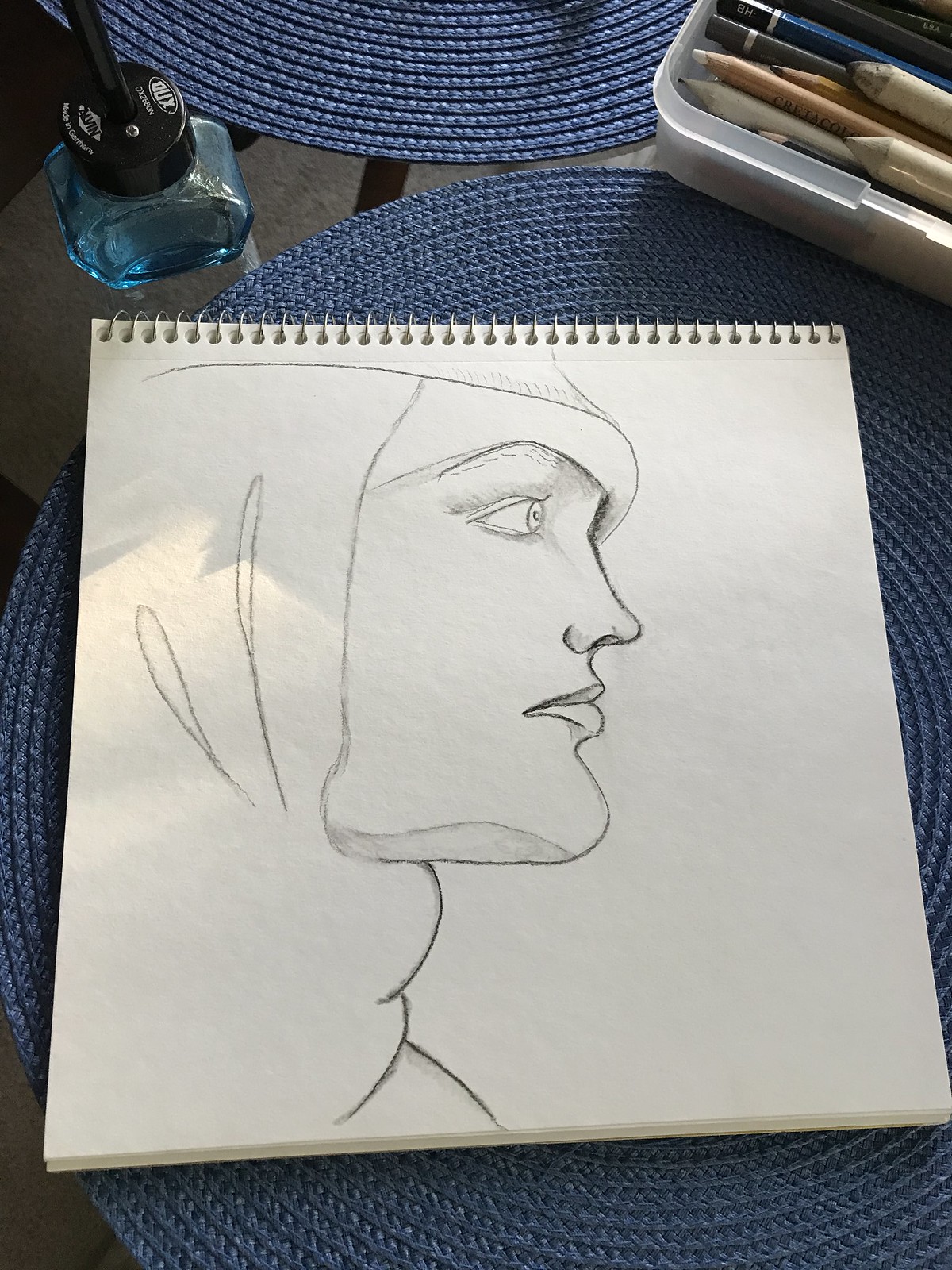This is a pencil sketch showcasing the intricate profile of a human face, captured with exceptional detail. The fine lines emphasize the delicate features of the lips, nose, eyes, and brow, revealing the artist's meticulous attention to detail. Subtle highlights under the chin add depth and dimension to the sketch. The subject appears to be adorned with a headdress or a knit cap, as evidenced by the textured lines around the edge of the head covering. Below, a few more lines suggest the presence of a shawl or scarf gracefully draped around the base of the neck. The sketch is drawn on a white spiral-bound sketch pad, which rests on a dark blue-gray knitted surface. In the upper left corner of the image, there is a dark blue bottle, possibly a perfume bottle, adding an element of contrast to the scene.